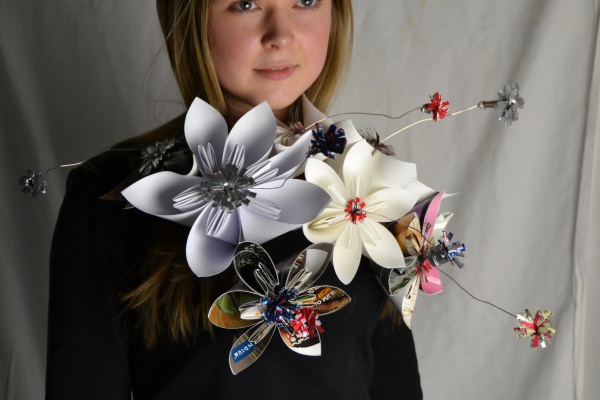The image features a teenage girl with long, dirty blonde hair draped over her shoulders, partially obscuring her face. She wears a black top, though it's unclear whether it's a long sleeve shirt or a dress as the image is cropped just above her waist. The backdrop appears to be a plain gray sheet. She is looking slightly off to the right. Across her chest, there is a striking arrangement of handmade flowers in various sizes and colors, primarily white, silver, gray, pink, and green. Some of these flowers seem intricately crafted from materials like magazines, with some featuring attached words, while others have long metal rods extending from them with small, shiny tassel-like flowers at the ends. The floral arrangement gives the impression of an artistic piece, suggesting creativity. The image appears to be taken indoors, with the girl standing directly in front of the gray backdrop, which further highlights the vivid and diverse floral embellishments pinned to her top.